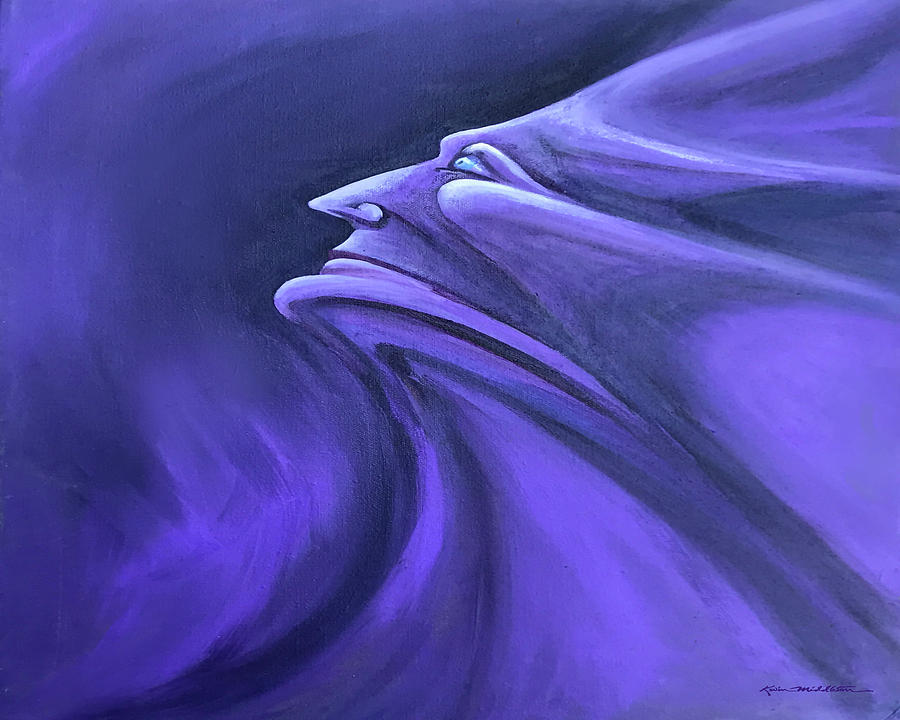The painting is a square-shaped, abstract artwork predominantly rendered in shades of blue and purple. Central to the composition is a tightly contorted face, seemingly pulled and stretched in a fabric-like manner that creates smooth folds and wrinkles suggestive of a tense, elastic material or wind swept effect. The face, characterized by blue eyes and a pointy nose, gazes towards the top left corner, with the defined nose pointing leftward. The mouth and chin are also discernible, with the entire visage exuding an emotion of fear. At the bottom right corner of the painting, the artist's signature is visible in black ink, adding a personal touch to the abstract yet profoundly expressive piece.